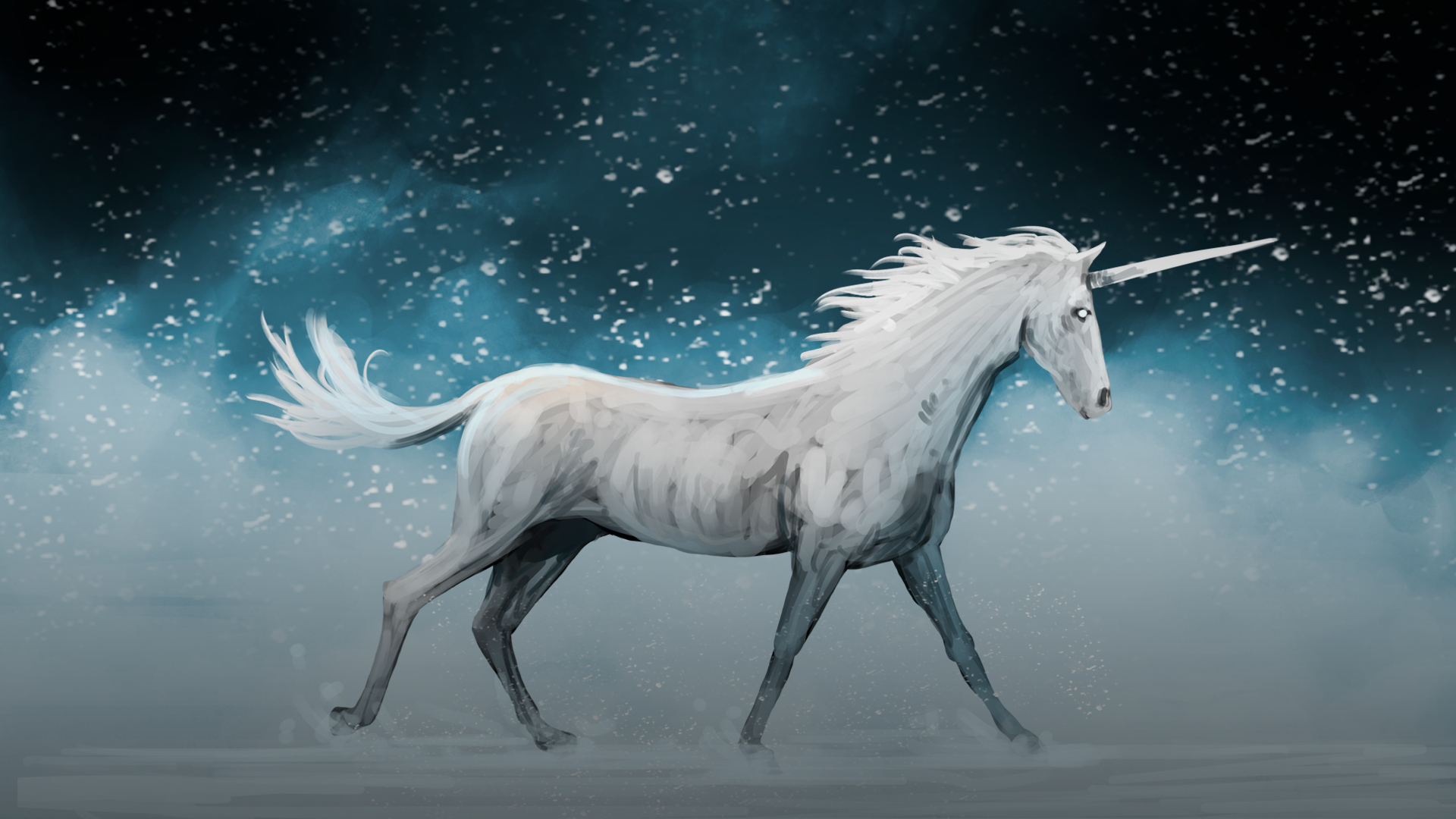The image is a highly detailed artistic depiction of a majestic unicorn, rendered with what appears to be wide strokes of paint, though it could also be a digital creation. The unicorn is completely white with a very long horn protruding from its forehead. It has a flowy white mane and tail, and its body is shown in a side view, walking or running through water, with droplets splashing up around its hooves. The unicorn's head is held high, exuding a sense of pride and strength, with a white glowing eye adding to its ethereal presence. The background is a dark sky filled with smoky white and blue dust, flecked with what appears to be falling snow or rain. This creates a stark contrast against the dark blue tones of the night sky, enhancing the unicorn's almost otherworldly glow. The ground also has a misty, smokelike white appearance, adding to the mystical atmosphere of the scene. The entire piece is captivating, with its skillful use of lines and colors creating a beautifully intricate and interesting work of art.